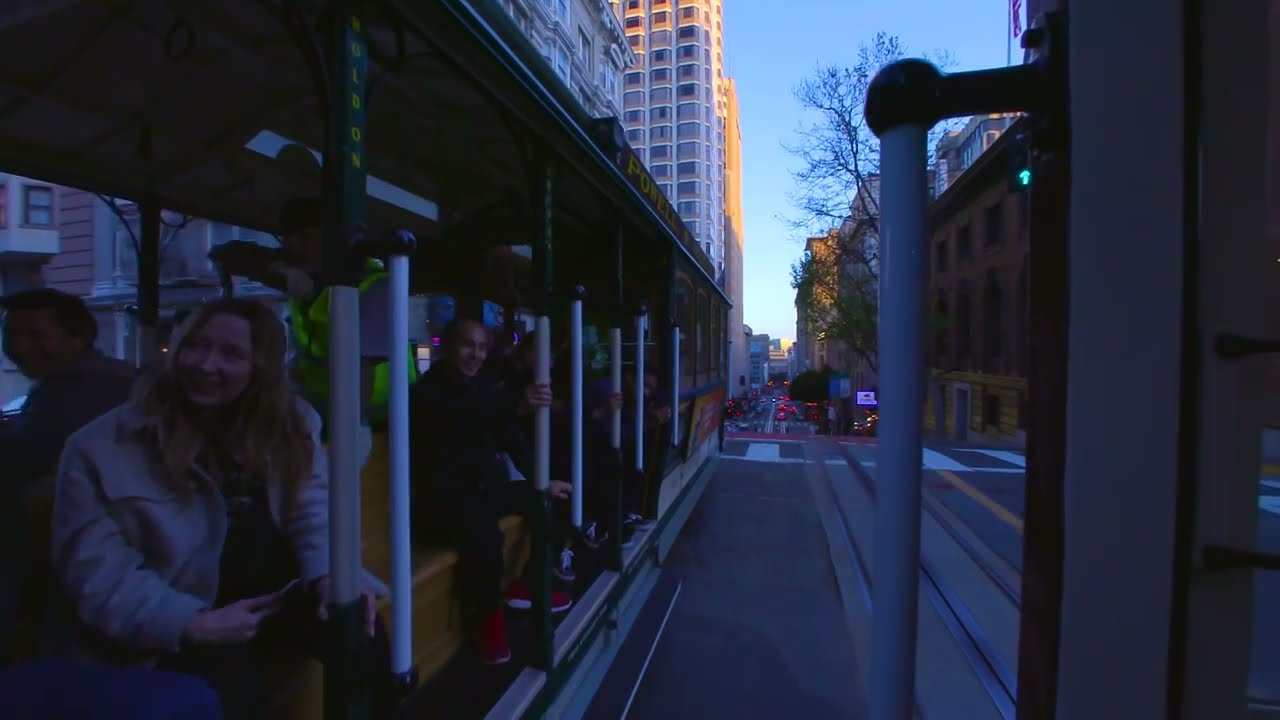The image depicts a bustling city scene at sunset, centered around a crowded trolley. People inside the trolley are either looking forward or glancing outwards toward the streetscape. The scene unfolds on a wide, city street that stretches into the horizon, flanked by high-rise apartment buildings with numerous windows. The street features a yellow-striped line running down its middle, and a few traffic lights in the distance signal "go" with a green light. On the right side, there is a tree with no leaves, suggesting it might be fall, alongside another tree that still has green leaves. A red building and other structures continue along the street, culminating in an overlook platform on the left side with steel posts, where several onlookers gather. A silver guardrail fronts this platform, and nearby signage, though illegible, adds to the urban atmosphere. Additionally, a second trolley, partially visible, shares the tracks, enhancing the sense of motion and transportation convenience in this cityscape.